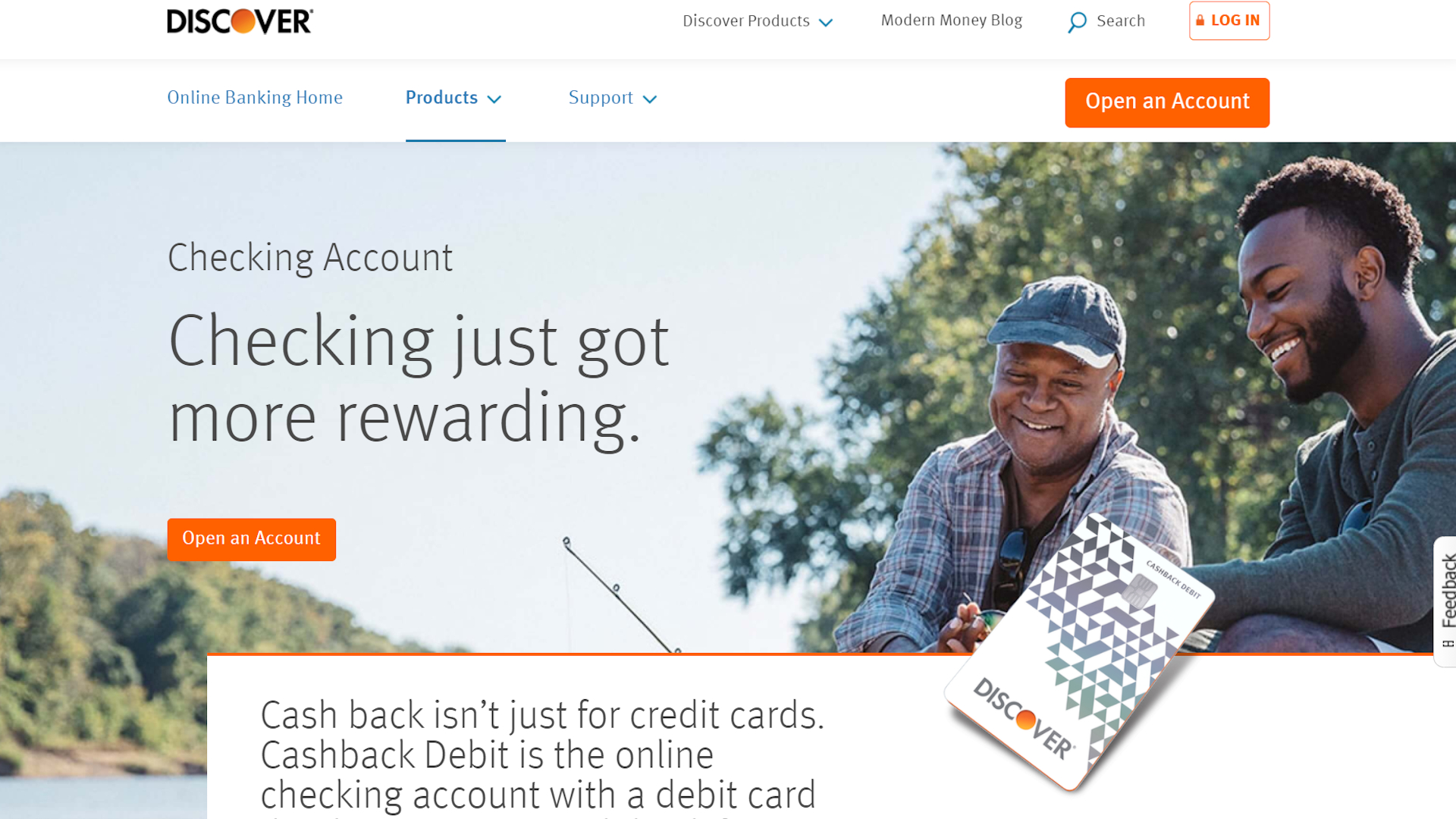The screenshot showcases a Discover website set against a pristine white background. In the upper left corner, the bold black Discover logo is prominently placed, with the 'O' uniquely represented as an orange circle. To its right, the navigation menu appears in a light gray font, listing options: "Discover Products" with a pull-down menu, "Modern Money Blog," and a small search bar. An action key labeled "Login," presented as a white button with orange text, sits beside another action button saying "Open an Account."

Below the header, there's a vibrant, outdoor photograph of two men engaged in fishing on a serene lake. Positioned in the upper right of the photo is a younger man, while an older man is seated below him, holding a fishing rod. The upper left corner of the image boasts a headline, "Checking Account," with the subtext, "Checking just got more rewarding." An additional orange action button reading "Open an Account" is situated towards the lower left of the image.

Below this, gray text on a white background reads, "Cashback isn't just for credit cards. Cashback Debit is the online checking account with a debit card."